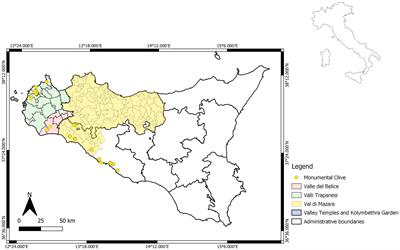This image displays a detailed map of a section of Italy, specifically focusing on Sicily. In the top right corner, there is a smaller outline of Italy for geographic context, with Sicily highlighted as the zoomed-in region at the tip of the boot. The main map itself is bordered by a black and white pattern and features multiple color-coded areas, including green, yellow, red, blue, and white, each representing different regions or attributes.

Most prominently, the map shows various valleys: green shading marks Valle Trapa, yellow shading represents Valle dei Mazziaria, red shading indicates Valle dei Belce, and blue shading identifies Valle Temelis, as per the legend on the right side. The legend also includes yellow dots denoting Monumental Olive trees and white lines for Administrative Boundaries. Additionally, there is a north arrow for orientation, and a scale bar that measures distances up to 50 kilometers, with the first 25 km shaded in black and the next 25 km in white.